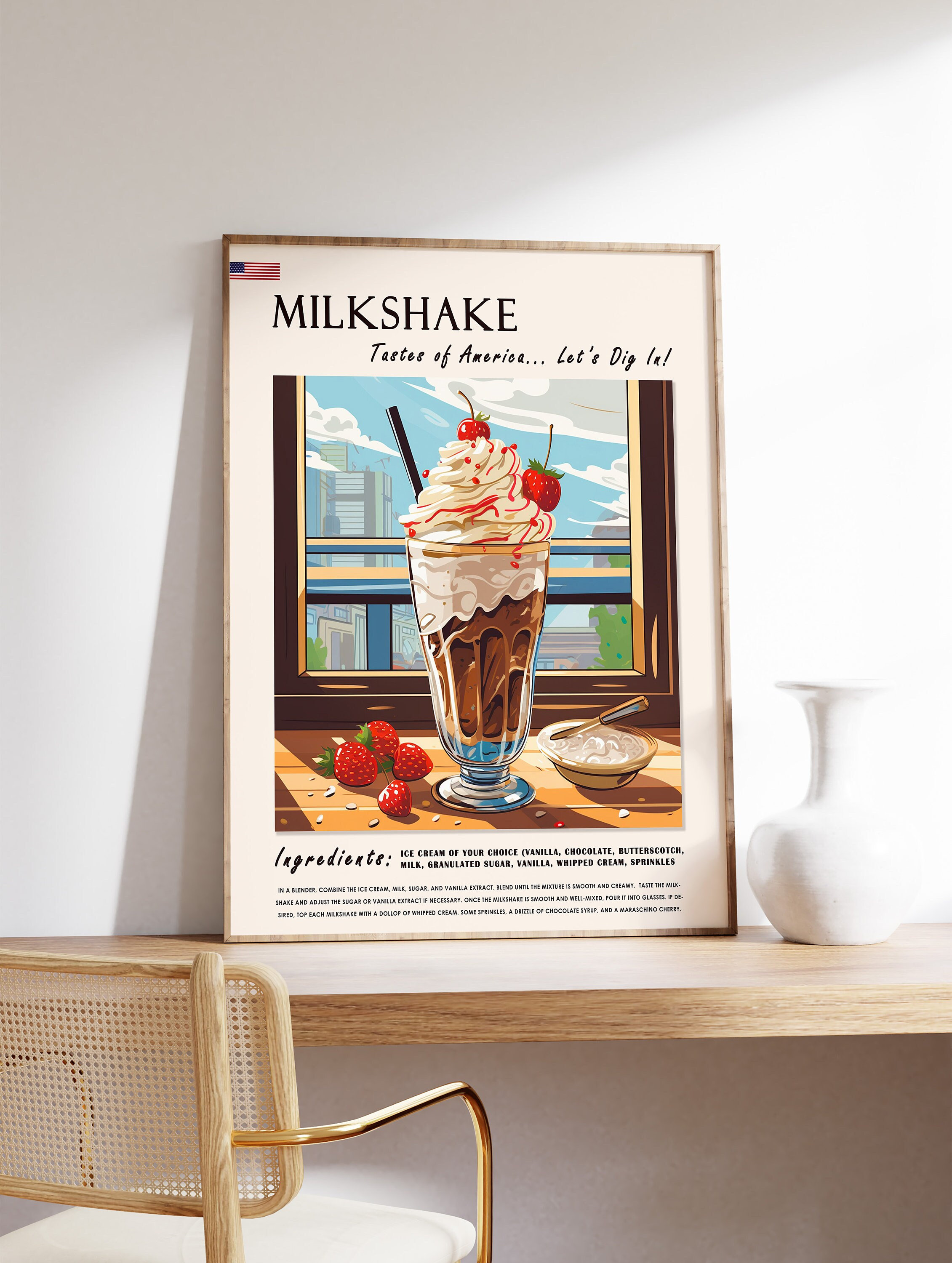This image showcases a serene room featuring a half-moon-shaped side table made of light beige wood that almost appears shelf-like due to its design. Resting on the table is an empty white vase. Positioned to the left of the table is a chair with a white base, light beige upholstery, and gold armrests. The central element in the room is a framed poster that leans against a white wall above the table. 

The poster vividly illustrates a chocolate and vanilla milkshake topped with whipped cream, strawberries, a cherry, and a black straw. This decadent milkshake is positioned on a wooden surface adorned with additional strawberries and a small bowl of whipped cream or butter accompanied by a butter knife. 

In the background of the illustration, a window reveals a blue sky dotted with white clouds and a cityscape. Above the milkshake, bold black letters read "Milkshake, Taste of America, Let's Dig In." Beneath the milkshake image, the word "Ingredients" precedes a detailed breakdown in very small print. The poster also features an American flag icon in the upper left corner.